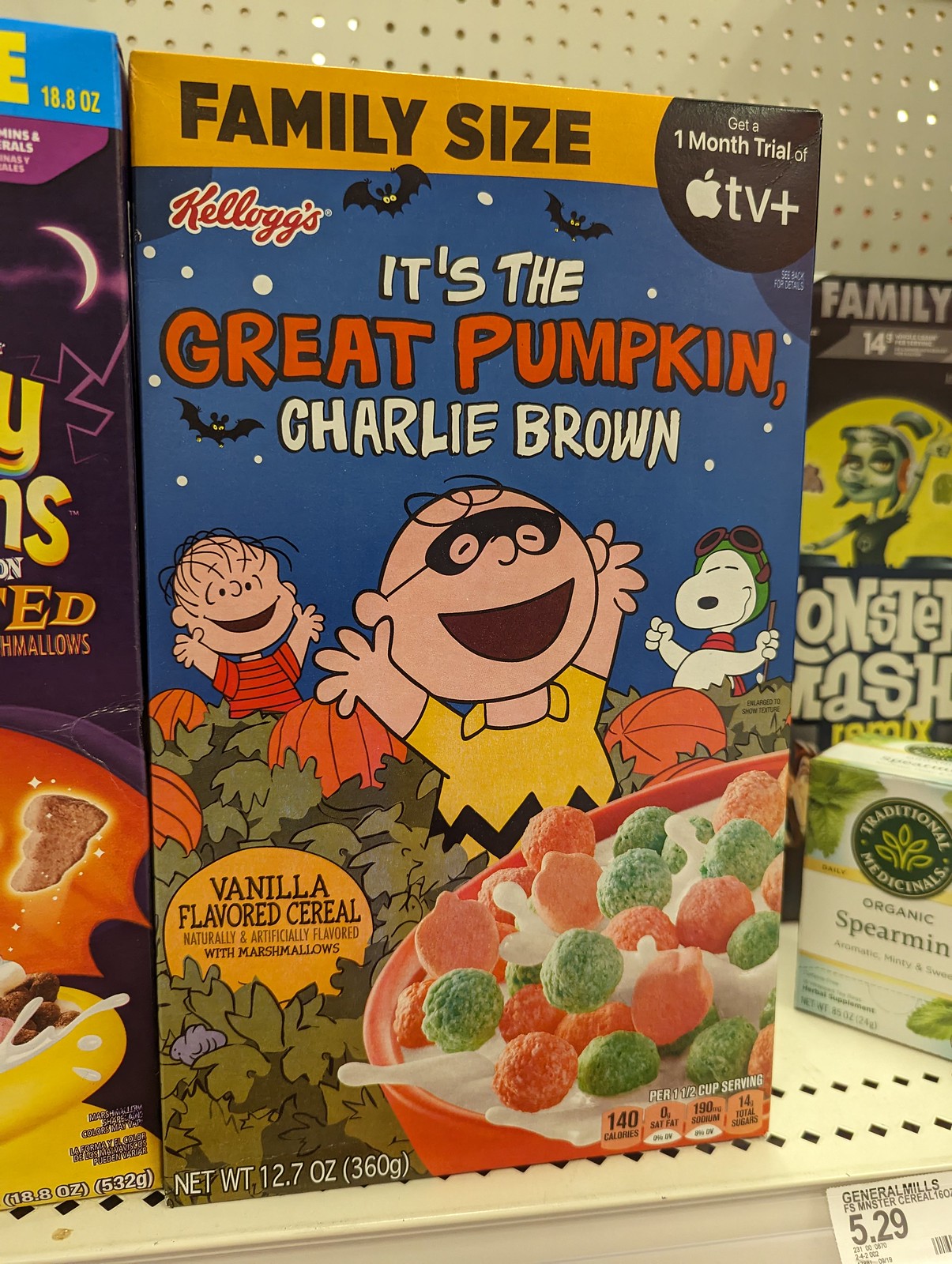Displayed prominently on a store shelf, this family-sized box of Kellogg's "It's the Great Pumpkin, Charlie Brown" cereal captures attention with its vivid imagery and nostalgic design. Priced at $5.29, as indicated on the bottom-right corner of the price tag, the cereal box features a joyful scene where Charlie Brown, Linus, and Snoopy are celebrating in a pumpkin patch filled with green leaves and large orange pumpkins that resemble basketballs. The trio stands with hands raised joyfully, against a backdrop of a dark blue sky dotted with tiny cartoon bats, evoking the playful and festive spirit of Halloween.

The top of the box proudly declares "Family Size," and just below it, in the upper left corner, is the Kellogg's logo. Centrally displayed on the box, the characters are highlighted, with Charlie Brown donning a Lone Ranger-style mask. To the right and left of him are Linus and Snoopy, respectively, all of them sharing the spotlight amidst the pumpkin patch. On the lower part of the box, there is a clear view of a bowl of the vanilla-flavored cereal, which is naturally and artificially flavored with marshmallows, described in the text below.

Adding a modern touch, the box includes an advertisement for a one-month trial of Apple TV Plus. Alongside the cereal box, smaller boxes, such as a box of Traditional Medicinal Spearmint Tea, are arranged neatly, making the bright and cheerful cereal box the focal point of this section. Additionally, the net weight of the cereal is specified as 12.7 ounces (360 grams), providing key product details for interested shoppers.